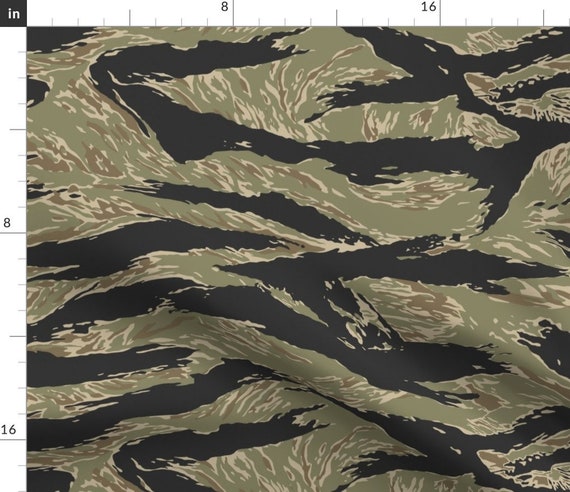The image showcases a detailed photograph of a fabric available for sale, designed to illustrate to customers the repetitive pattern and precise measurements, with inch markers along the left and top borders ranging from 8 to 16. The fabric features a bold yet muted camouflage design or animal print that is reminiscent of zebra or tiger stripes. The pattern is composed of artistic, textured brush strokes and abstract forms, with colors predominantly in dull olive green, interspersed with shades of off-white, brown, light beige, and dark gray or black. This creates an illusion of waves or rolling hills, adding depth and dimension to the fabric, giving it a sense of textured peaks and valleys. The black patches, reminiscent of tiger stripes, contrast sharply against the more subdued background colors, forming a striking and visually complex design.